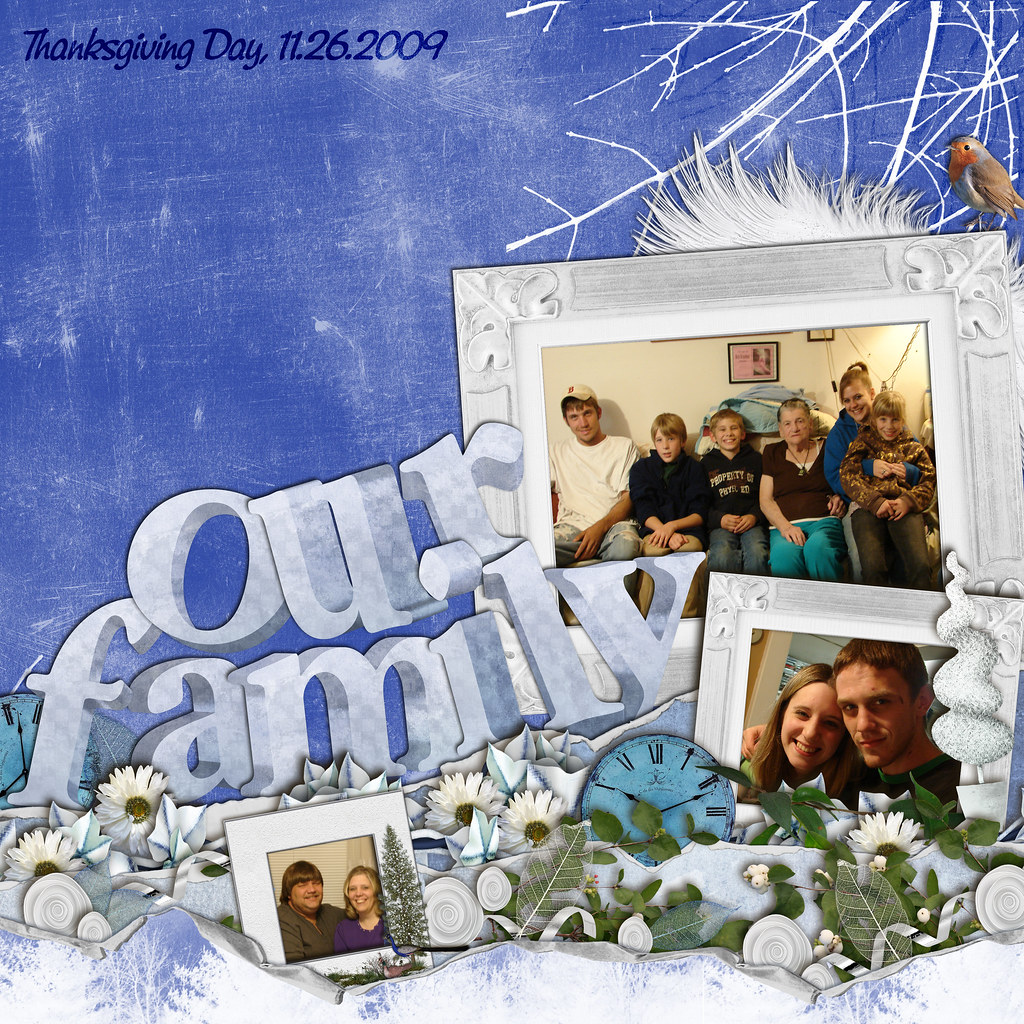The image appears to be a digitally designed Thanksgiving card dated November 26, 2009. The background imitates a frosty or icy day and is decorated with snowy branches and white picture frames, along with a drawing of a robin perched on the top photo frame. In the top left corner, blue text reads "Thanksgiving Day 11-26-2009" and beneath it, in large letters, "Our Family."

The largest picture is on the right-hand side, showing a family of six: two adults, three children, and an elderly woman. The adult male is wearing a white t-shirt, and there are two boys in black hoodies. The elderly woman and an adult female are present, with the latter having a child on her knee. The family appears to be smiling and acting goofy while seated on a chair.

Below this main picture, there is a smaller image of a couple; the man has medium-length brown hair, and the woman is blonde and wearing a purple top. To the right of the main image is another small photo of a man with short brown hair and a blonde woman, possibly in their late teens or early twenties. The man looks directly at the camera with a slightly unsettling expression, while the woman is smiling.